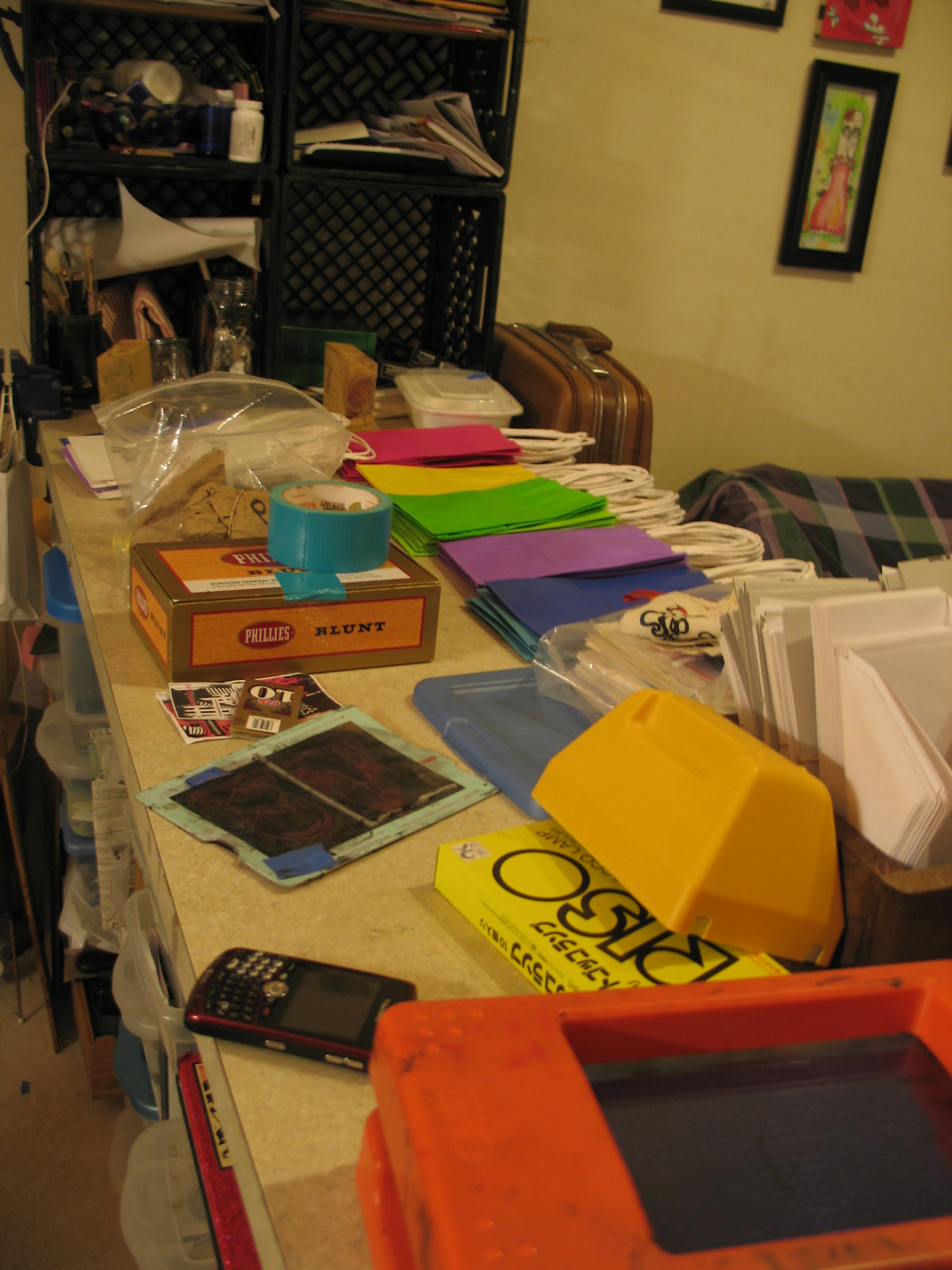A cluttered and chaotic room, possibly serving as an art studio or creative space, is depicted in the image. Central to the scene is a large plywood table, ornately cluttered with colorful storage bags in vibrant hues of pink, yellow, lime green, purple, and blue. In the background, a bed or couch is partially visible, adding to the room's multifaceted use. The table also hosts a collection of envelopes and a conspicuous cigar box, haphazardly sealed with blue duct tape.

Adding to the disarray are several gray-black plastic milk crates, overflowing with scattered papers, contributing to the overall messy ambiance. A vintage BlackBerry phone lies inconspicuously amongst the clutter. On the floor near the milk crates, a well-worn brown suitcase completes the scene. The entire setting evokes a sense of disorganization and creative chaos, leaving the viewer slightly uneasy.